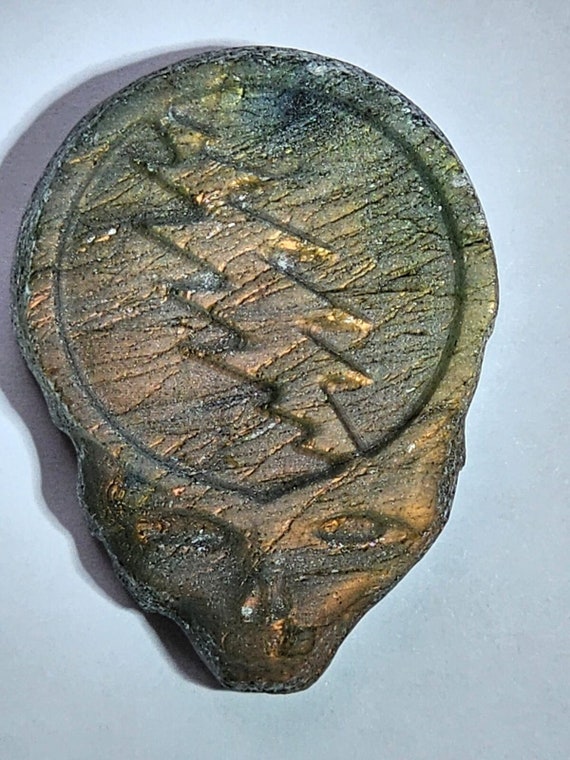The image depicts a color photograph, shot in portrait orientation, looking down from an overhead perspective at a peculiar object situated against a light gray background. The object appears to be a wooden carving or potentially an ancient artifact, with a skull-like face featuring distinctly hollow eye sockets and a pointed chin at the bottom. The carving has a flattened, circular top that sports a raised, diagonal lightning bolt pattern extending from the upper left to the lower right. The overall texture and color of the object is a mix of gold, gray, copper, and green hues, resembling aged wood or pottery. The deep indention and small raised rim around the perimeter heighten its three-dimensional quality, accentuating its alien, otherworldly appearance.